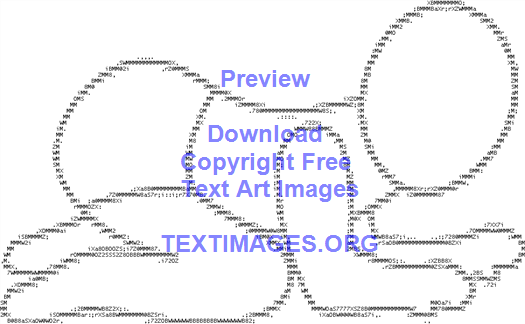The image is a computer-generated drawing of what appears to be a crawling infant or a person in a kneeling position, made entirely of tiny, black text characters. These characters include random numbers, letters, and punctuation marks, outlining the extremities such as arms, legs, and thumbs. Interestingly, the thumbs on the right hand are positioned where the pinky would normally be. The body of the figure is composed of intricate text, and while the detailed head is present, it lacks a face. The interior of the image remains white, contrasting with the dense text outline. Overlaid across the center in easier-to-read blue text are the words: "Preview, Download, Copyright Free, Text Art Images," and a website link, "textimages.org." This text watermark suggests that the image serves as an advertisement for a business providing text art images.